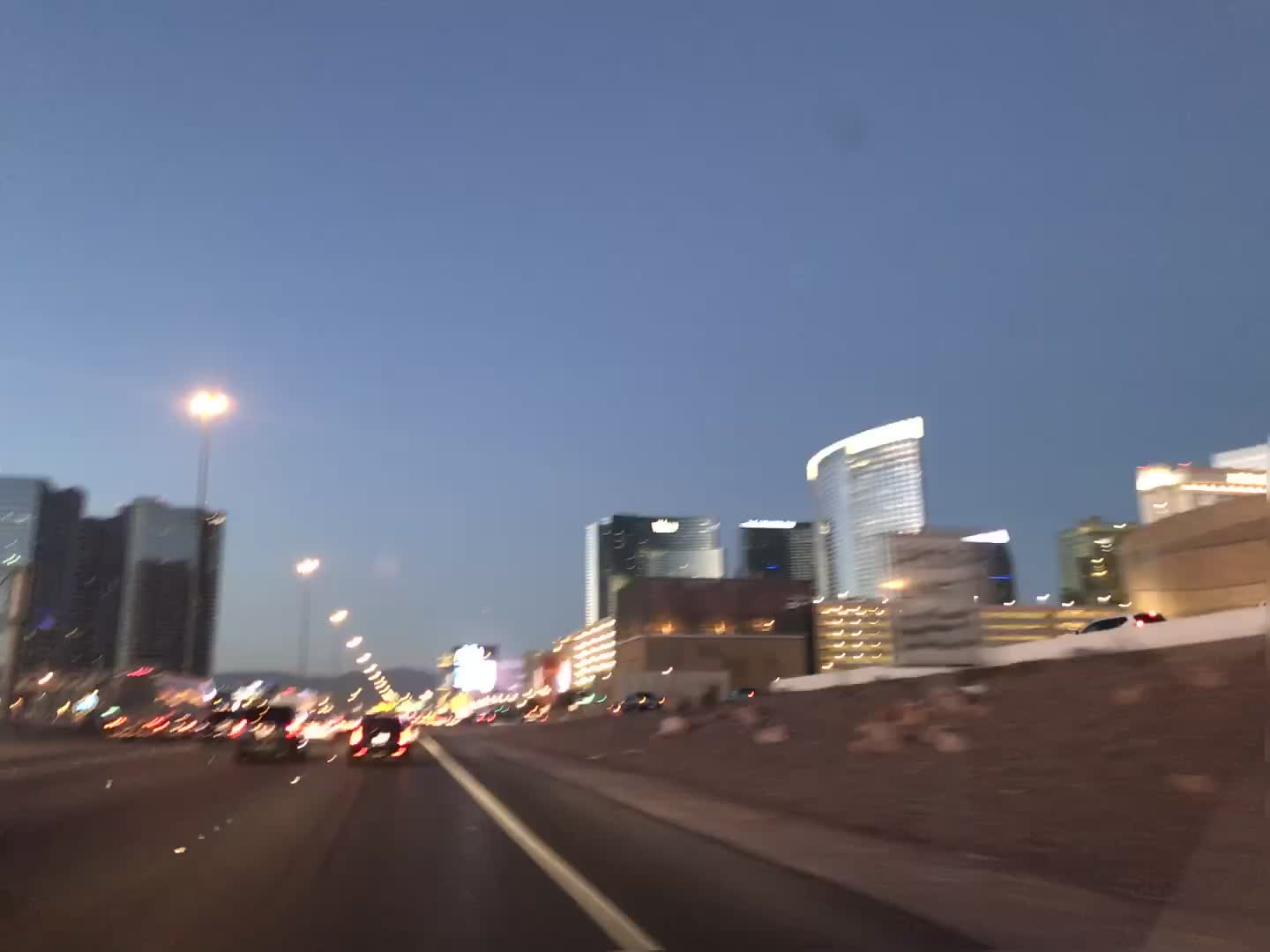This blurry photograph captures the bustling atmosphere of a downtown scene as viewed from an interstate highway with four or five lanes. On the right, a concrete barrier separates the lanes, and blurred taillights and headlights of vehicles indicate the busy traffic. To the left, a couple of towering buildings dominate the skyline, while on the right, four notable structures are visible. Among them, one stands out with an oval shape, and another resembles a parking garage. The photo also captures a merging lane where vehicles are entering the flow of traffic, suggesting the presence of an on-ramp. The scene is set during twilight, with the sky still holding onto the last light of the day. This image encapsulates the dynamic and fast-paced environment typical of urban settings at dusk.